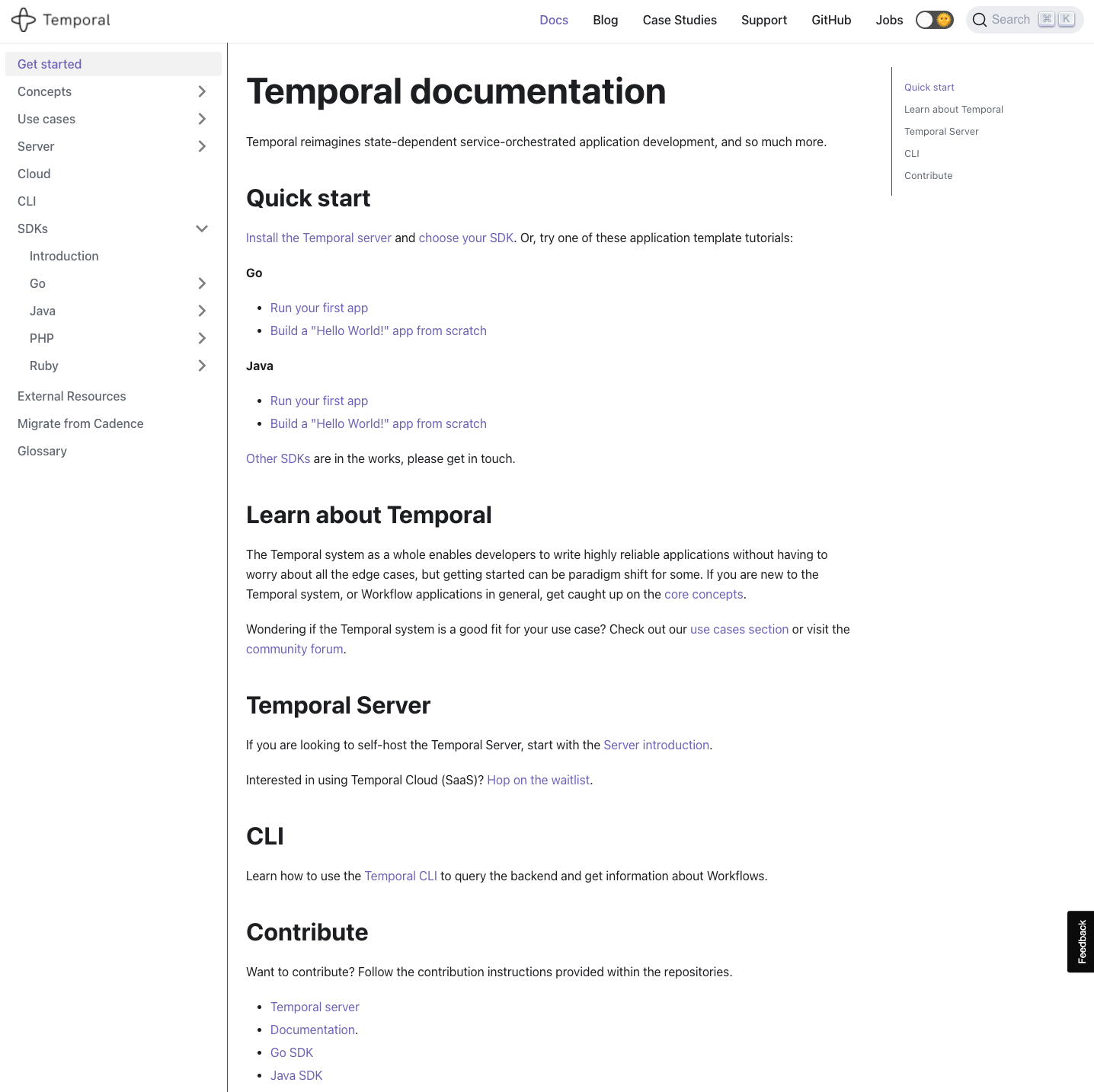This is an interface for a website dedicated to the software product called Temporal. Prominently displayed at the top is the name "Temporal," accompanied by a small plus sign. Directly below is a navigational menu featuring the options: "Get Started," "Concepts," "Use Cases," "Server," "Cloud," "CLI," "SDKs," "Introduction," "Go," "Java," "PHP," "Ruby," "External Resources," "Migrate from Cadence," and "Glossary," all arranged along the left side of the interface.

The central section features a header labeled "Temporal Documentation," with subheaders detailing the product's capabilities, including "Temporal Reimagined," "State Dependent Service Orchestration," and "Application Development." Further below are quick access links for "Quick Start," available in both "Go" and "Java," as well as sections to "Learn About Temporal," the "Temporal Server," and "CLI." At the bottom of this section is a link labeled "Contribute."

The layout is designed to provide comprehensive information about the Temporal software, aiding users in everything from initial setup to advanced feature utilization and community contributions.